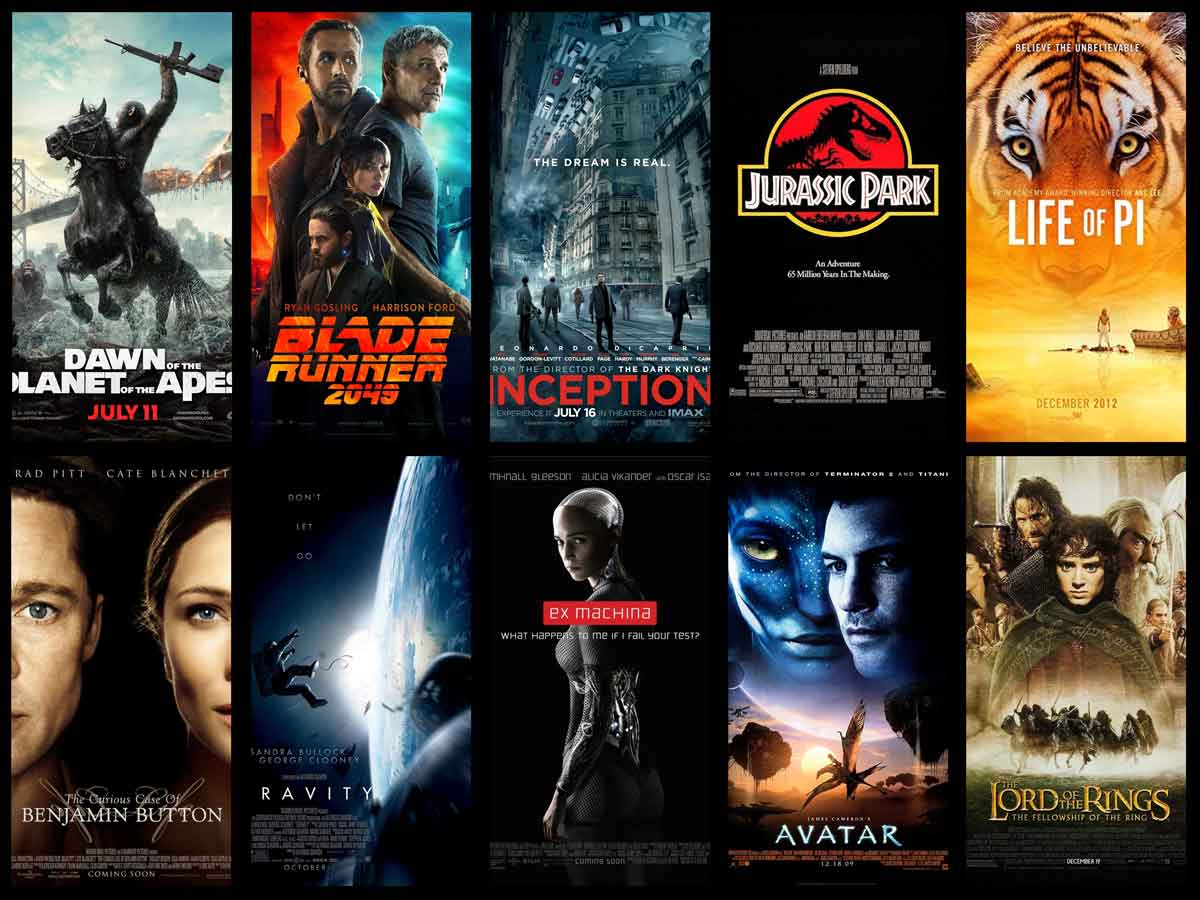The image is a photo collage of 10 vibrant movie posters, organized in a grid with 2 rows and 5 columns. Each poster is a vertical rectangle and is framed by a thin black border, enhancing the visual separation. The top row, from left to right, features posters for "Dawn of the Planet of the Apes," "Blade Runner 2049," "Inception," "Jurassic Park," and "Life of Pi." The bottom row, from left to right, includes posters for "The Curious Case of Benjamin Button," "Gravity," "Ex Machina," "Avatar," and "The Lord of the Rings: The Fellowship of the Ring." Each poster contains a compelling image and the title of its respective movie, contributing to the colorful and neatly arranged display set against a black background.